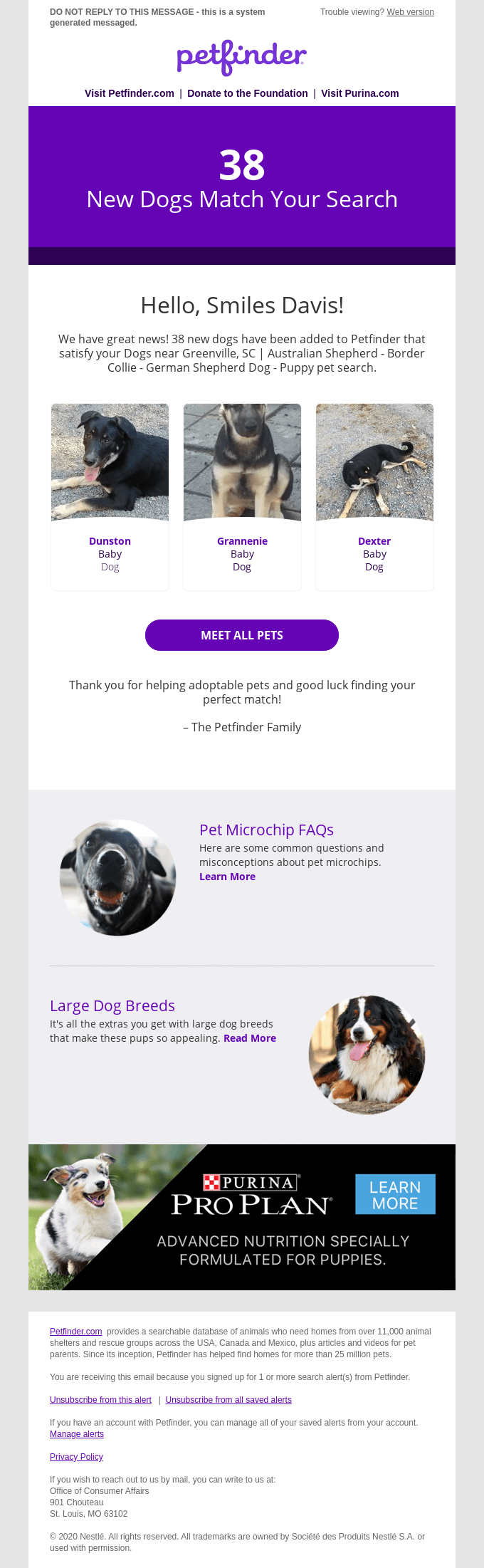In this detailed image displayed on an Android phone screen, the header reads "Do Not Reply to This Message" in all caps, followed by a note that this is a system-generated message, although some text is blurred. The interface prominently features "Petfinder" in lowercase, cursive purple text. Below this, a link and a call to action urge the viewer to visit petfinder.com and donate to the foundation.

Further down, there is a reference to Purina Lotus and some user information, possibly "hello smiles Davis.” The main section includes a centered paragraph, flanked by three images of dogs, with the central dog appearing to be a German Shepherd. An oval, purple button labeled "View All Pets" is visible underneath these images.

On the left, the section titled "Pet Microchip Facts" includes a few lines of text and a "Learn More" link. Below this area is another section titled "Large Dog Breeds", which presents two paragraphs followed by a purple "Read More" link. Adjacent to this section, "Purina Pro Plan" is highlighted with a blue "Learn More" button next to an image of a dog. This last section promotes enhanced nutrition specially formulated for puppies, accompanied by additional informational text.